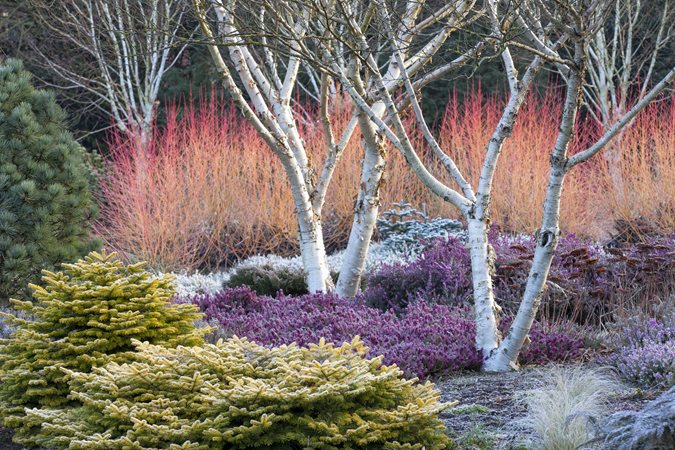In this vibrant and compelling outdoor photograph, three small, barren trees with striking white bark stand prominently in the center against a tapestry of rich, diverse plant life. The ground is a mosaic of low shrubs and bushes, with a light green shrub in the foreground, a purple, heathery looking shrub at the center, and a tall, fiery orange and red shrub in the background that almost appears ablaze. Surrounding these focal points is an expanse of various greenery, punctuated by a few scattered rocks. Despite the natural setting, the photograph's elements seem to possess varying light qualities, as if captured from different moments or adjusted to achieve a unique, composite effect. The overall scene, devoid of visible dirt and marked by well-defined details, exudes a serene yet surreal ambiance, suggesting a carefully curated depiction of nature.